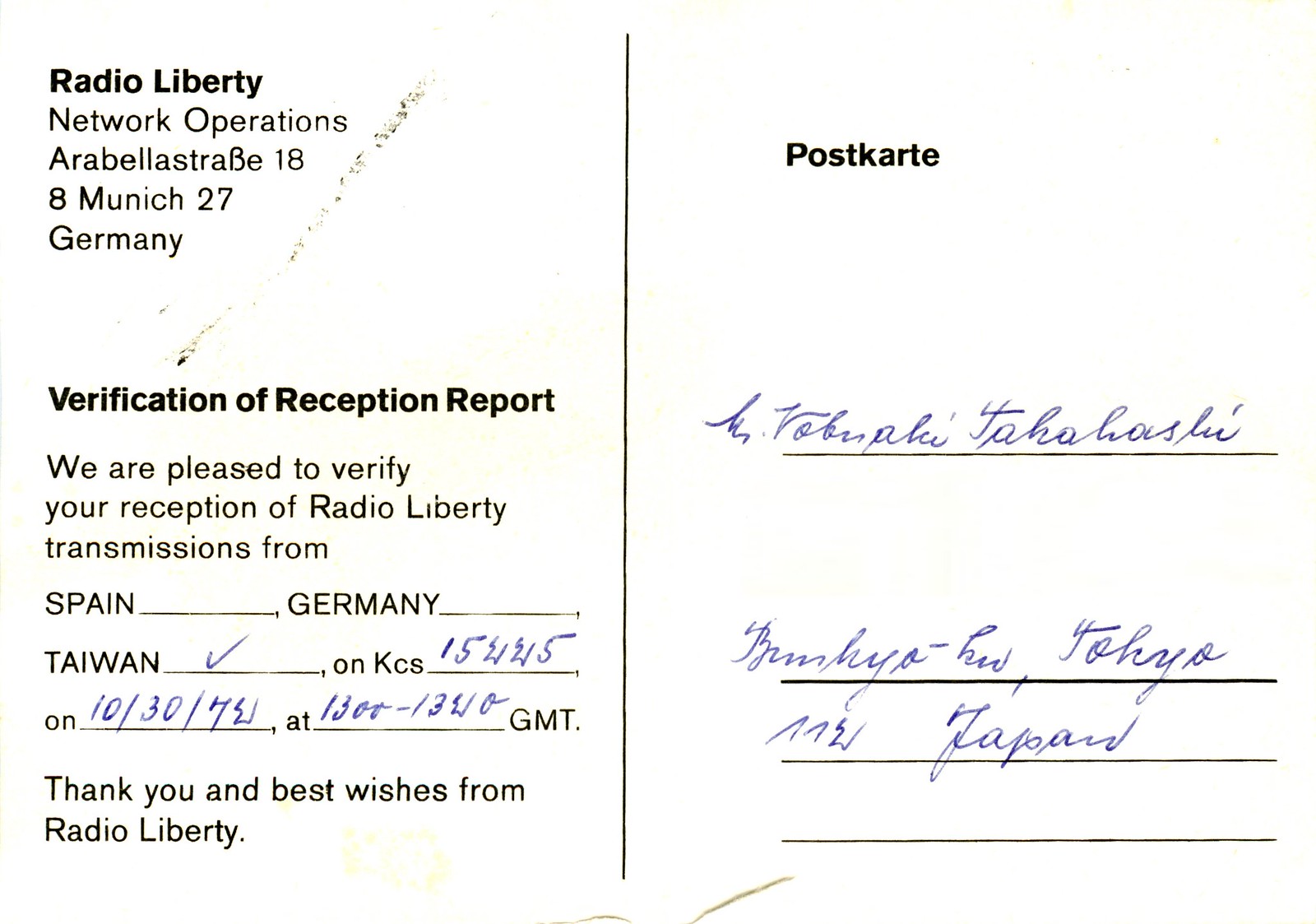This horizontal, rectangular postcard features a white background with black text, and several details are filled in with blue pen. On the left-hand side, the text reads: "Radio Liberty Network Operations, Arabella Strasse 18, 8 Munich, 27 Germany." Below that, it says, "Verification of reception report," followed by, "We are pleased to verify your reception of Radio Liberty transmissions from Spain, Germany, and Taiwan." Next to Taiwan is a blue checkmark. The frequency "KCS 15,445" and the date "10/30/74" at "1300 to 1340 GMT" are handwritten in blue pen. The message ends with, "Thank you and best wishes from Radio Liberty." 

A vertical black line divides the postcard, with the right side labeled "Postcarta." There is an illegible handwritten name and address in a foreign language, but "Tokyo, Japan" is discernible. Additional horizontal black lines beneath the handwriting suggest a format for an address.